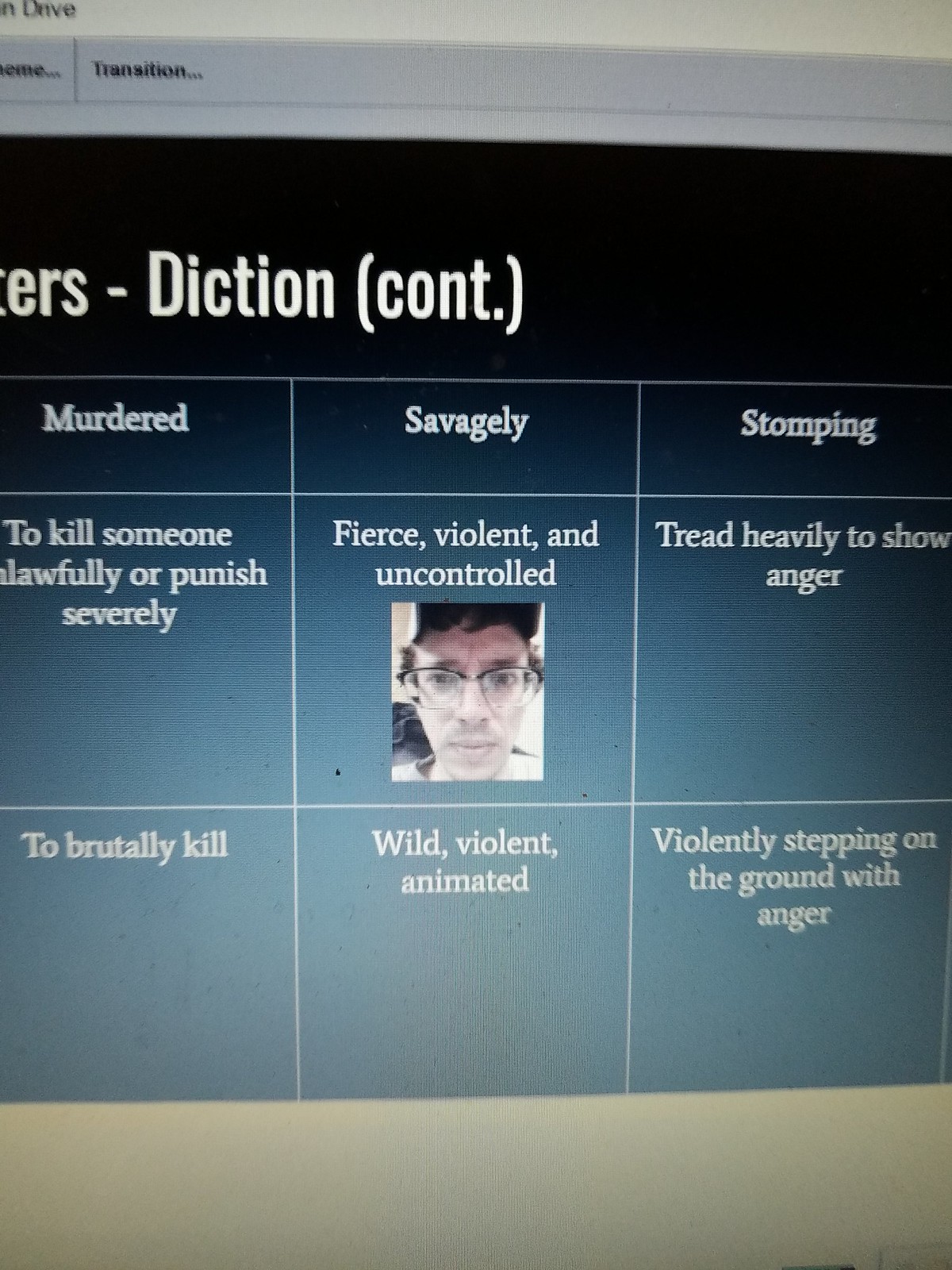This image captures a computer screen displaying a chart against a gradient blue background, titled "Transition..." at the top within a grey header. The chart features three columns labeled "Murdered," "Savagely," and "Stomping," each with detailed definitions over two rows. Under “Murdered,” the definitions read "to kill someone unlawfully or punish severely" and "to brutally kill." The "Savagely" column defines it as "fierce, violent and uncontrolled," and includes a photograph of a young white man wearing glasses, with the description "wild, violent, animated." The "Stomping" column specifies "tread heavily to show anger" and "violently stepping on the ground with anger." Above the chart, text reads "diction (continued)," indicating the continuation of an explanation.